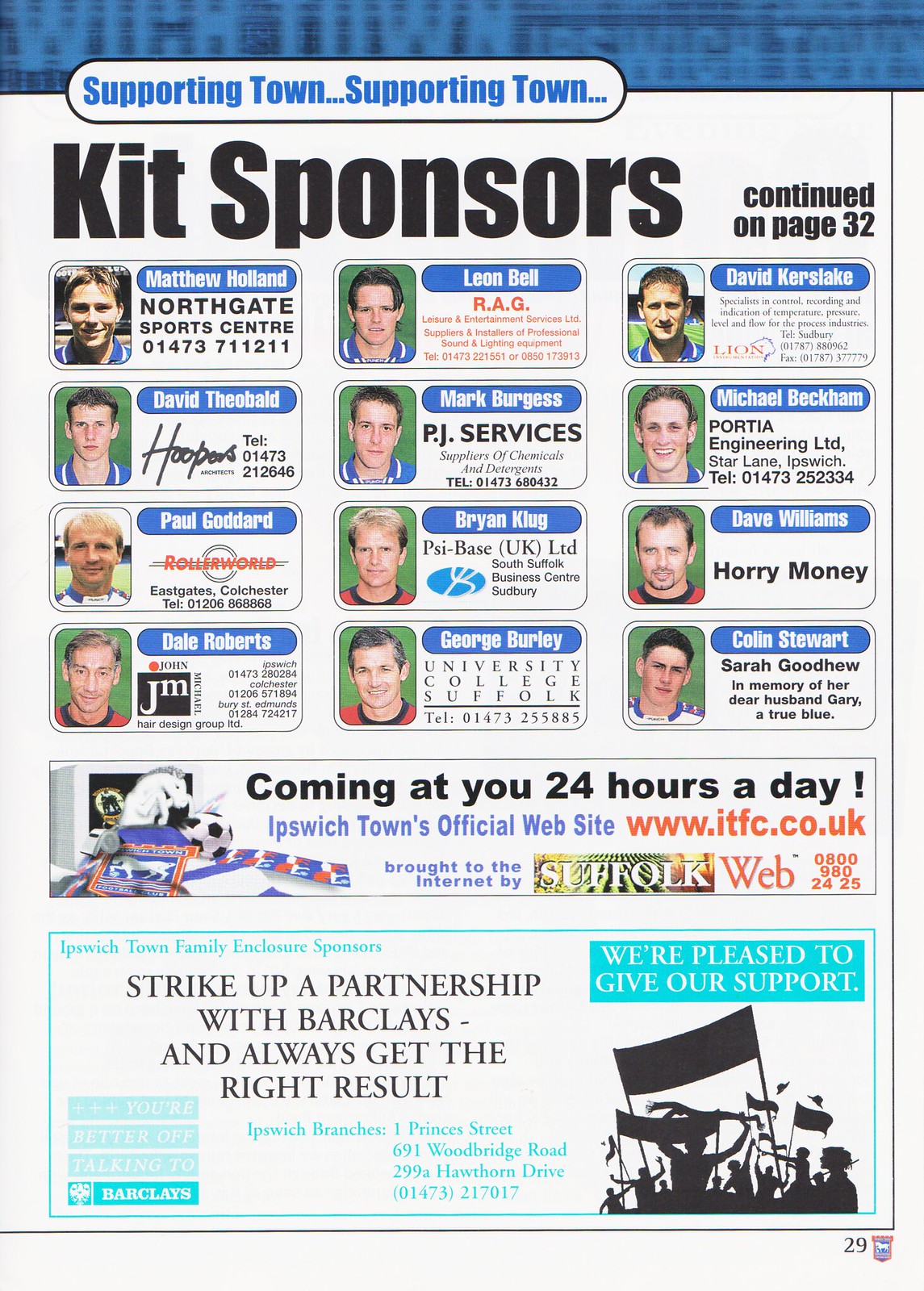The image is a magazine page featuring several advertisements related to a sports team. At the top is a white poster with a rounded blue tab inscribed in blue lettering, "Supporting Town, Supporting Town." Just below in large, black text, it reads, "Kit Sponsors, continued on page 32." Beneath this heading, there are 12 black-outlined rectangles, each containing a headshot of a light-skinned man with their respective names placed in blue labels with white lettering. The names listed are Matthew Holland, Leon Bell, David Kerstake, David Theobald, Mark Burgess, Michael Beckham, Paul Cotterd, Brian Klug, Dave Williams, Dale Roberts, George Burley, and Colin Stewart. Alongside each individual’s name and image, there are affiliations with varied companies or educational institutions. 

Below this section, spanning the width of the page but occupying only about an eighth of the page height, there is another advertisement with a white background and black font that states, "Coming at you 24 hours a day, Ipswich Town's official website," along with the URL, "www.itfc.co.uk." 

At the bottom of the page, there’s a final advertisement in aqua blue and black text reading, "We’re pleased to give our support. Strike up a partnership with Barclays and always get the right result," accompanied by a logo or silhouette image.